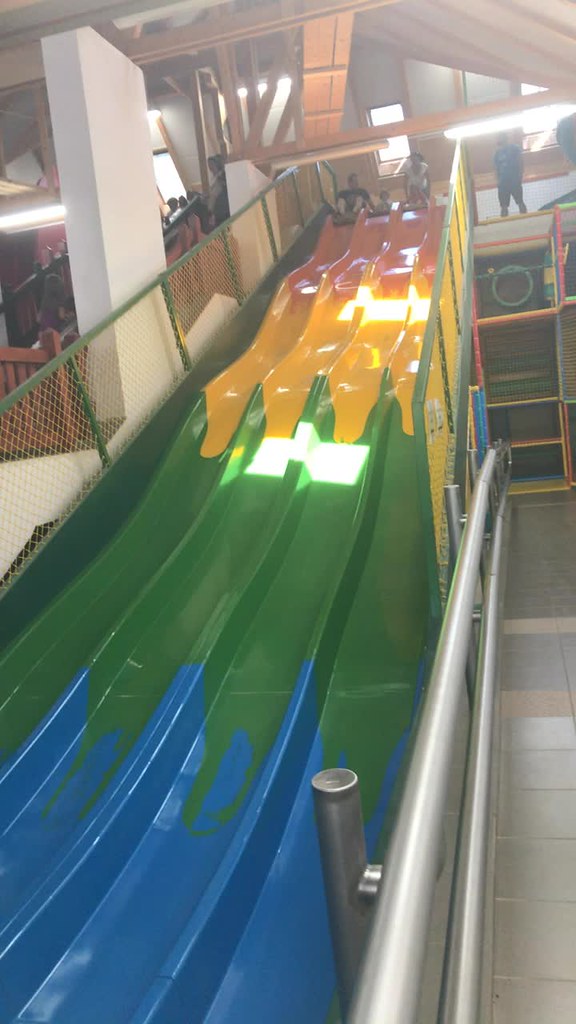This photograph captures a vibrant indoor recreation area featuring a towering four-person slide. The slide is a colorful gradient, transitioning from blue at the bottom to green, yellow, and finally red at the top. At the summit, a family of three—a father in the leftmost lane, a child in the second lane, and a mother in the third—sits on slide mats, ready to descend. Next to them stands a staff member supervising the activity. The slide's structure includes distinct lanes separated by bridges, preventing cross-over between sections. Surrounding the slide, there are other play features, including a green pipe and a knitted climbing area. There are also steps and a metal railing leading up to the slide, with several people ascending. The ground is covered in tiling, and patches of sunlight filter through windows, illuminating different parts of the slide.